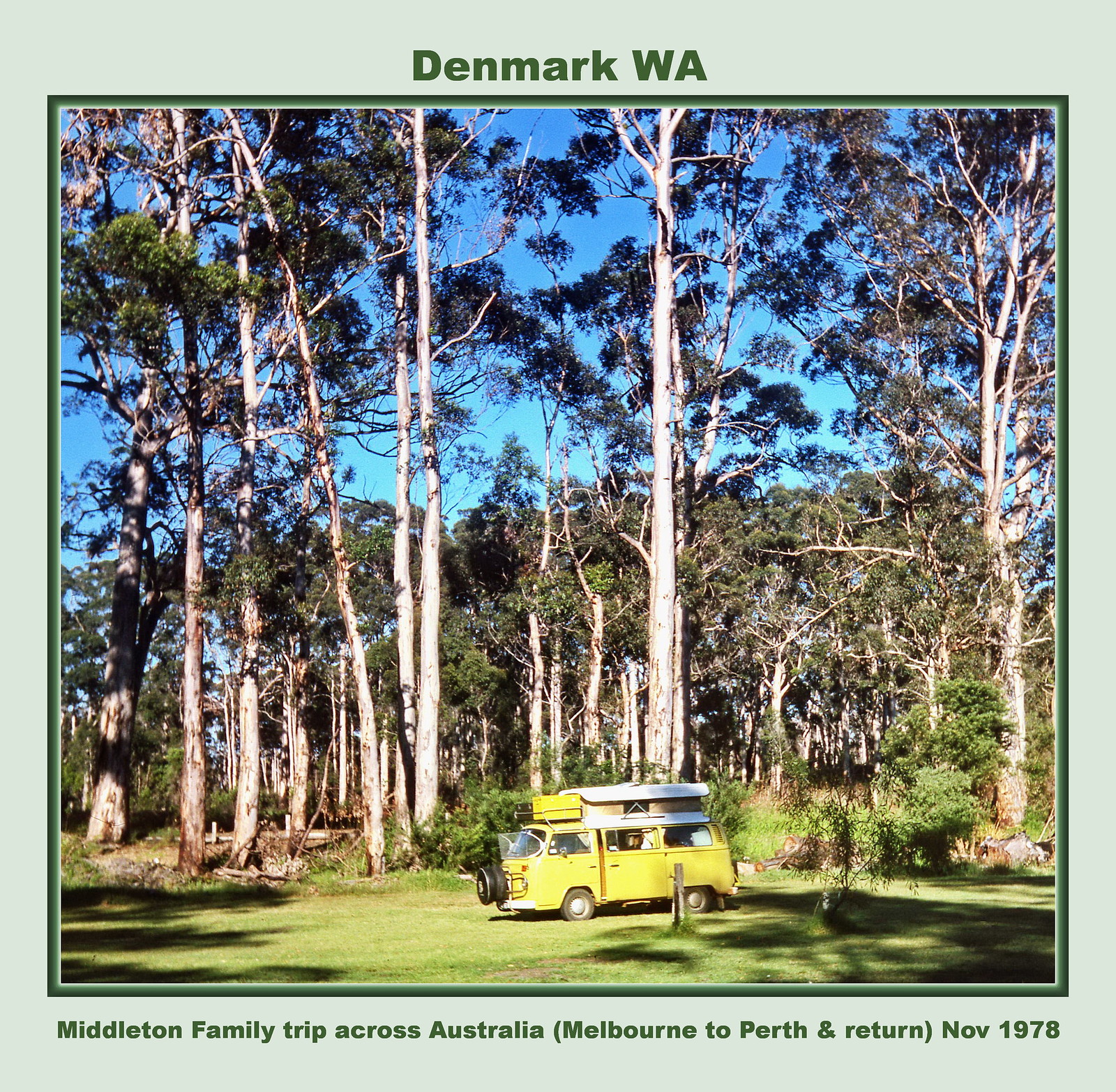The image is a colorful photograph of a bright yellow or possibly pea-green vintage van, reminiscent of an old Scooby-Doo style vehicle, parked on a lush plot of short grass. The van, equipped with camping gear and luggage on its roof, is set against the backdrop of a dense forest comprised of very tall trees with smooth, white trunks and sparse lower branches. Above the scene, the clear blue sky stretches out, indicating it's a sunny day. A caption in green text at the top of the image reads, "Denmark, W.A.," while the bottom contains another green text caption that states, "Middleton family trip across Australia," followed by "Melbourne to Perth and return, November 1978." Surrounding the photograph is a thin white and green border, framing this nostalgic and serene moment from the past.